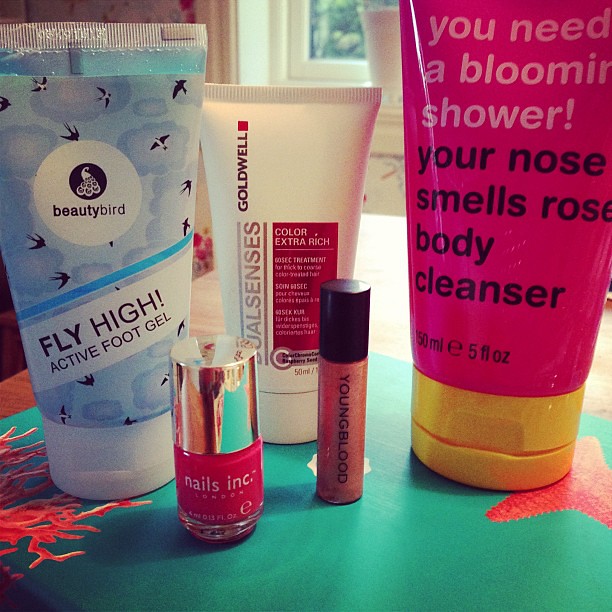The photograph, taken indoors with sunlight streaming through a window, showcases a variety of cosmetic products arranged on a turquoise-blue table adorned with an orange starfish and coral. Prominently featured in the background are three vertical tubes with flat flip-top caps: the leftmost tube, which has a blue cloud scene with birds and is branded "Beauty Bird," contains Fly High Active Foot Gel; the central tube, predominantly white with red accents, is labeled "Dual Senses Color Extra Rich" by Goldwell, suggesting it's for hair coloring; and the rightmost tube, pink with white and black text, reads "You Need a Blooming Shower – Your Nose Smells Rose" body cleanser. In the foreground, a bright pink nail polish container and a small, likely mascara product in a similar pink shade are positioned on the left and right respectively. The final item in the collection is a tube labeled "Youngblood," possibly containing bronzer. The scene captures a colorful and detailed display of beauty products in a vibrant and decorative setting.